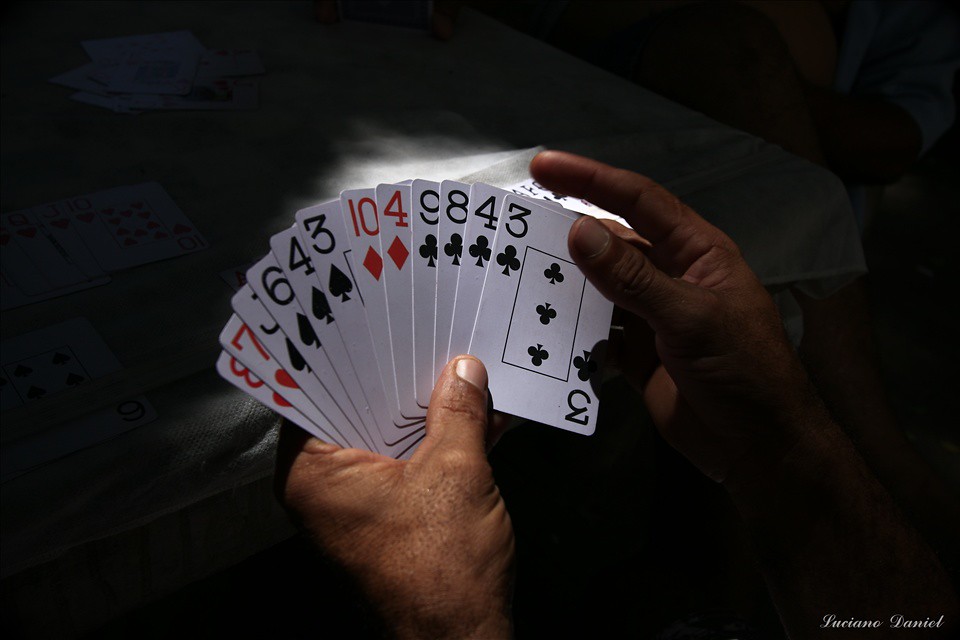This photograph, watermarked with the artist's name at the bottom, features a moody, black background with a subtle photo overlay effect. Resting against this backdrop is the soft, sunlit scene of a white tablecloth adorned with scattered playing cards. A pair of heavily wrinkled, weathered hands — likely those of an elderly man — are prominently placed in the foreground, holding a deck of cards with focus and intent. The visible cards in his hands include a three of clubs, four of clubs, eight of clubs, nine of clubs, four of diamonds, ten of diamonds, three of spades, four of spades, six of spades, jack of spades, seven of hearts, and eight of hearts. Behind these hands, on the table, additional cards can be discerned: a ten of hearts, jack of hearts, and queen of hearts are among the identifiable ones, while other cards remain indistinct. The scene is enriched by the interplay of light and shadow, with black shadows casting a dramatic effect over the man's hands, emphasizing the textures and depth of the image.